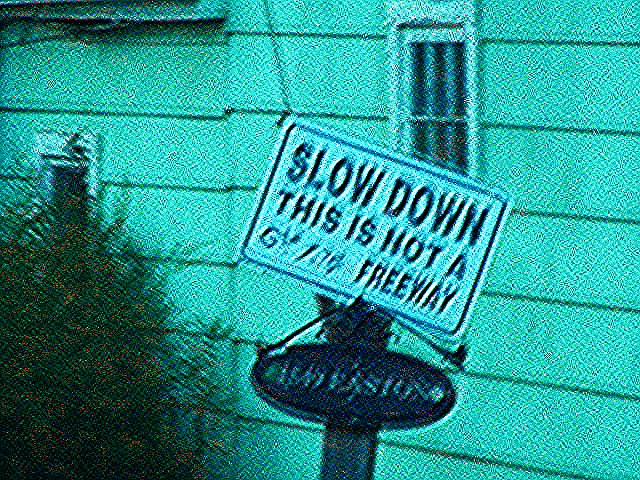The grainy image, likely captured by a closed-circuit camera, centers on a slightly crooked white street sign. The sign, marred by distortion, reads, "Slow Down, This is Not a... Freeway." Beneath it, a darker sign with faint light text appears to display a street number and the partially legible word "Easton." This sign arrangement is set against a light-colored house with wood or vinyl paneling and a thin window. To the left, partially obscured by distortion, stands a tree or shrubbery, with one or two power lines running through the background.